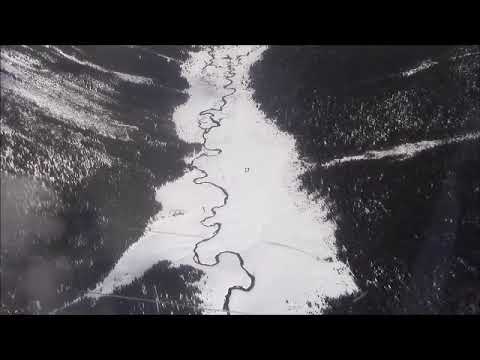The image is displayed inside a horizontally oriented rectangle with black borders on the top and bottom. It predominantly features a dark gray and charcoal black surface that serves as the background, which is interspersed with various white streaks and dots. Dominating the middle of the composition is an extensive white mass, appearing almost cloud-like, which runs from the top middle of the image and widens as it descends. Within this broad white area, a pronounced squiggly black line meanders from the top to the bottom, bisecting the white space. There's also a noticeable white appendage jutting out to the left near the bottom. The upper left corner contains faint white streaks slanting downwards, and there are similar streaks on the right side of the image, adding to the textured appearance. The overall aesthetic resembles a weather map or possibly an ultrasound image, giving it a nebular, almost ethereal quality.